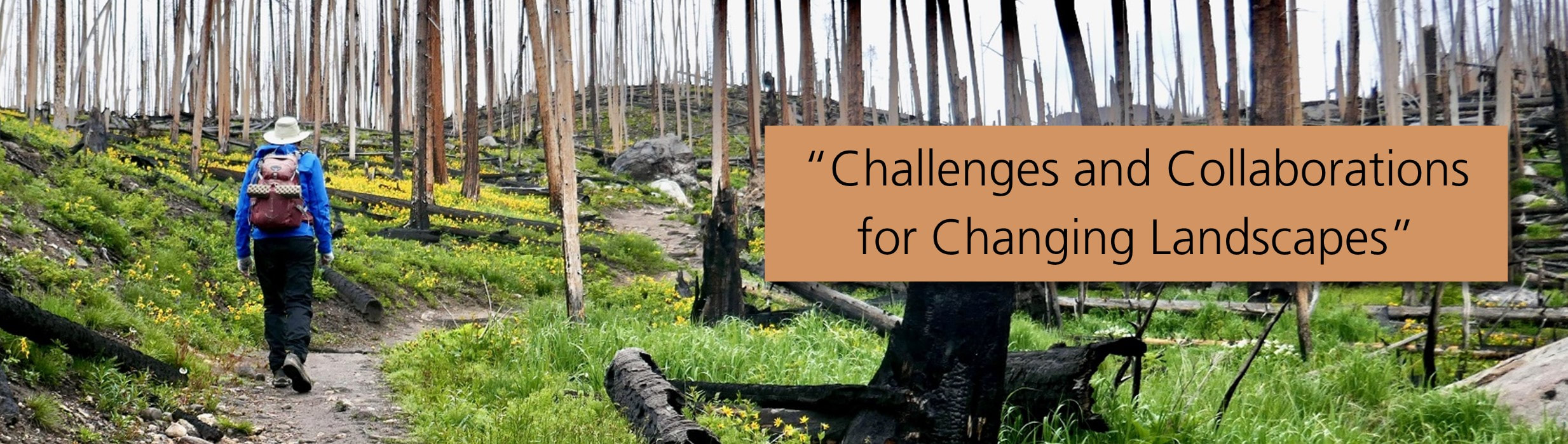In this wide, short photograph, approximately an inch and a half tall by six inches wide, a man is seen walking down a dirt path set in a barren, denuded hillside. He is dressed in a white cowboy-style hat, a blue jacket with a hood, dark blue or black cargo pants, and gray hiking shoes. He carries a red or off-pink backpack. The path is surrounded by sparse, bare trees stripped of their foliage and branches, resembling thin wooden posts. Fallen logs are scattered on the ground, adding to the desolate atmosphere. On either side of the path, grass and small yellow flowers grow, while a large rock juts out from the hillside. Above the image is an orange rectangle with black lettering that reads, "Challenges and Collaborations for Changing Landscapes."